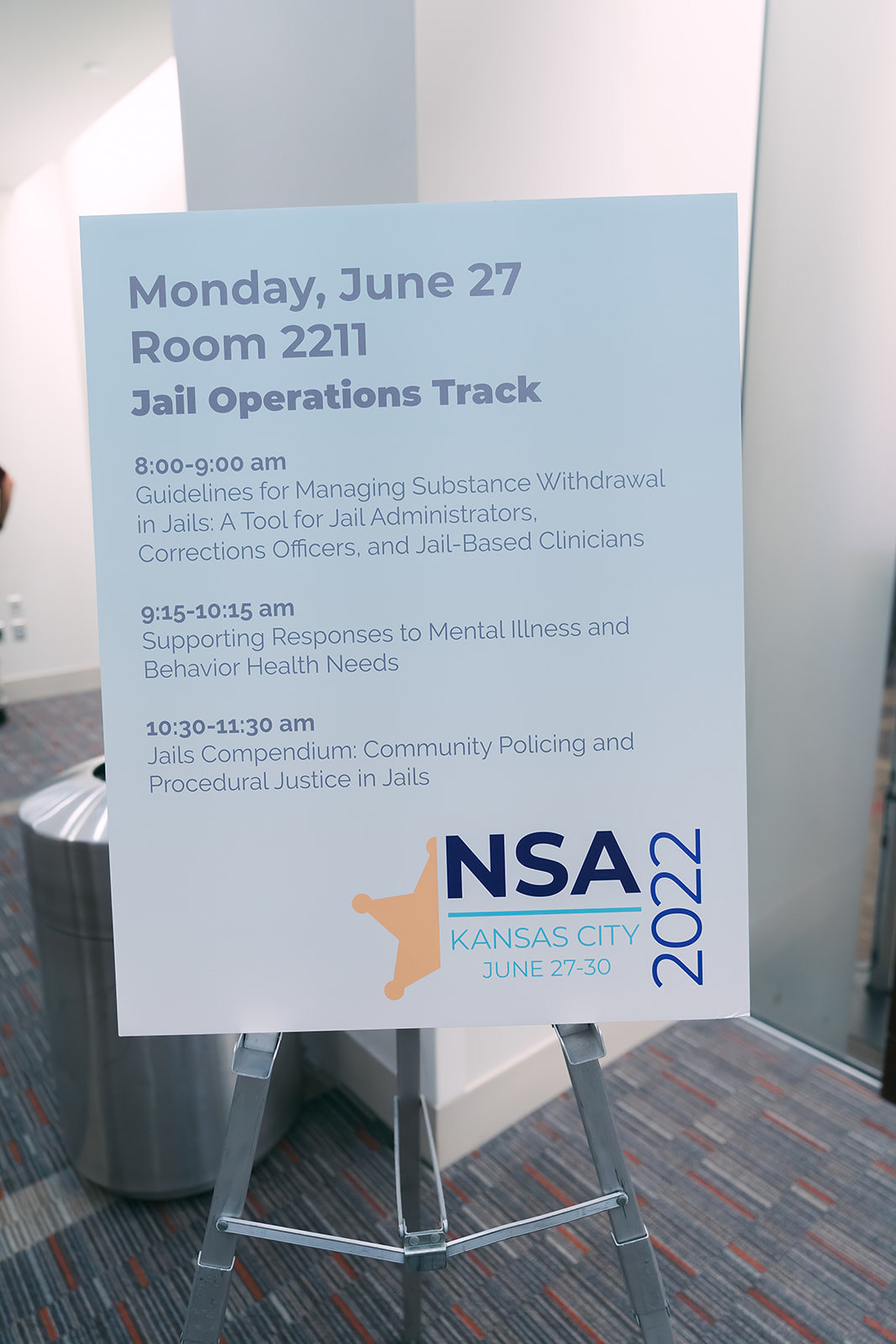The photograph shows a light blue banner with a turquoise gradient towards the bottom, positioned on a silver tripod. The banner details a schedule for a conference session taking place on Monday, June 27th, in Room 2211, focusing on the Jail Operations Track. The sessions are listed as follows: from 8 a.m. to 9 a.m., "Guidelines for Managing Substance Withdrawal in Jails: A Tool for Jail Administrators, Corrections Officers, and Jail-Based Clinicians"; from 9.15 a.m. to 10.15 a.m., "Supporting Responses to Mental Illness and Behavioral Health Needs"; and from 10.30 a.m. to 11.30 a.m., "Jails Compendium: Community Policing and Procedural Justice in Jails." The bottom right of the banner features a partially visible sheriff's star logo and the NSA logo, with "Kansas City, June 27-30, 2022" written in turquoise capital letters. The scene is set in a brightly lit office or conference hall with white or beige walls, a striped gray, red, and white carpeted floor, and a silver metal trash can visible in the background.